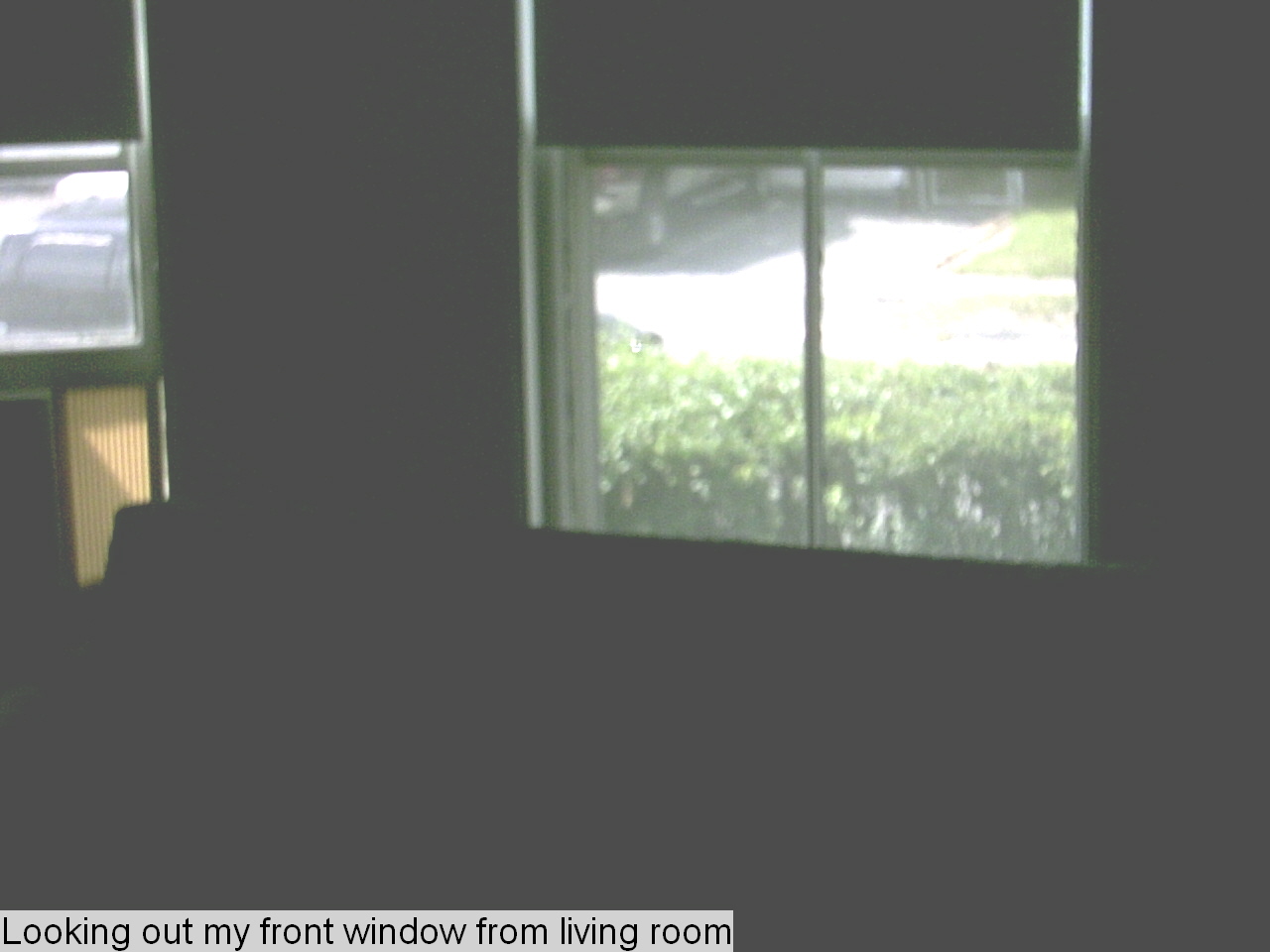The image portrays a view from a living room window labeled with the text "looking out my front window from living room" in black letters on a light grey square situated at the very bottom left. The primary focus is the window positioned centrally, featuring two vertical frames. The exterior scene appears sunlit, revealing green bushes immediately outside and further beyond, a greyish road or parking lot is visible. A car is parked to the left. The window has light shimmery grey sides, and below it is a yellow, ribbed structure framed in dark grey to black. Much of the screen is dark, contributing to a shadowed indoor atmosphere. Inside the living room, the walls are a medium dark grey, with a television mounted on the left wall. The television is on, surrounded by a black frame, but its content is indistinct. The photo overall has a slightly blurry quality with muted colors.